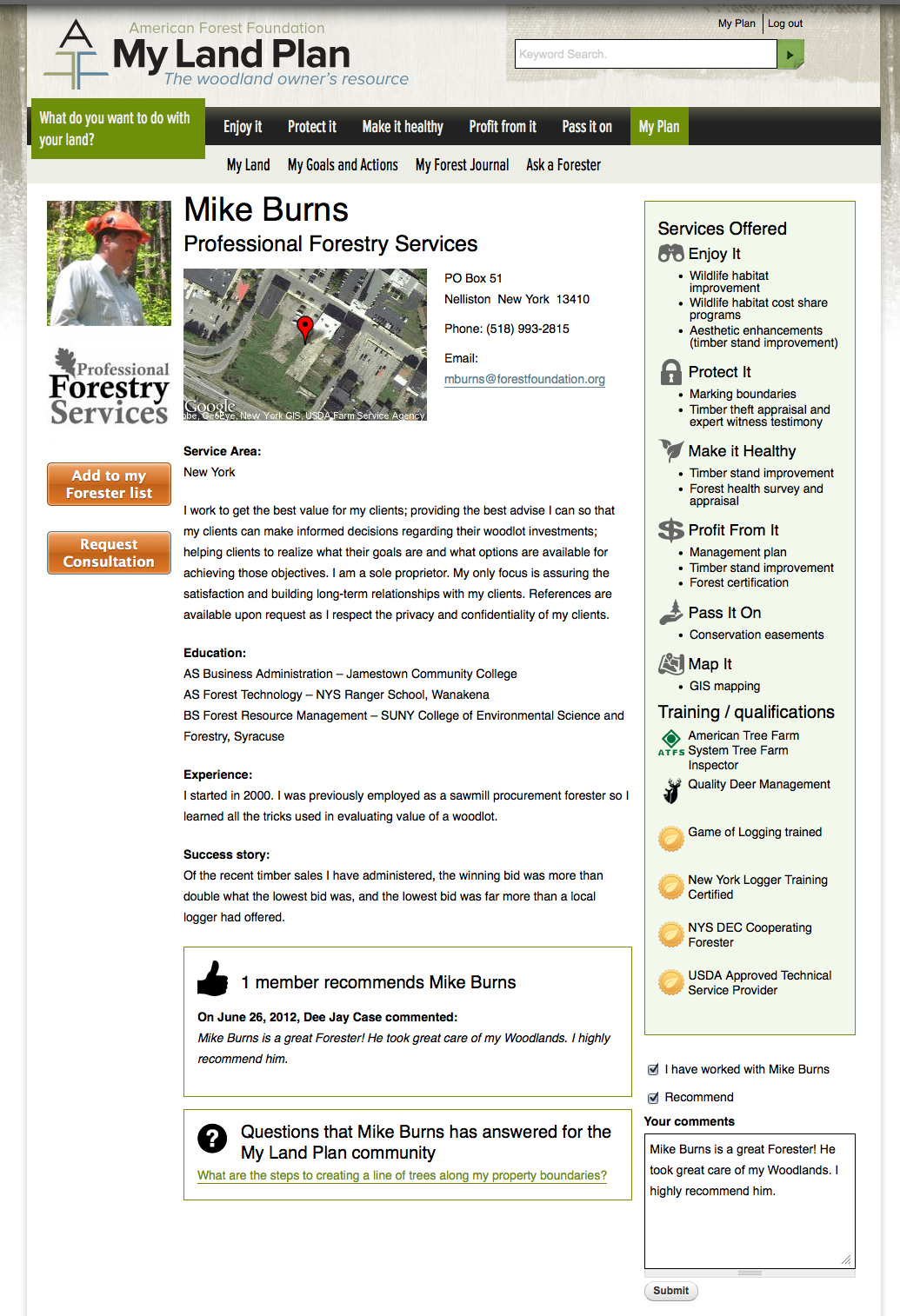The webpage from the American Forest Foundation's "My Land Plan" platform displays a wealth of resources for woodland owners. At the top of the page, there is a search bar, along with navigation options such as "My Plan" and "Logout." The central focus is on helping landowners determine their goals, with the prompt, "What do you want to do with your land?"

Highlighted prominently is Mike Burns and his professional forestry services. A map with a red dot marks his location, and contact details are provided, including a PO Box 51 in New York, along with his phone number and email address. His service area is outlined, and there are sections detailing his education, experience, and success stories. A thumbs-up icon indicates that one member has recommended his services, and there's a section listing questions Mike has answered for the "My Land" community.

On the left-hand side, there's a photograph of a man in an orange hard hat standing in a dense forest. This image is labeled "Professional Forestry Services." Below the image, users can either add Mike Burns to their forester list or request a consultation through clickable buttons.

The services offered by Mike include "Enjoy It," "Protect It," "Make It Healthy," "Profit From It," "Pass It On," "Map It," and "Training and Qualifications."